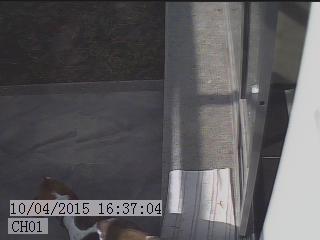This image is a bit challenging to interpret due to its small size and low lighting. The scene appears to be indoors, perhaps viewed through a security camera or something like Ring. The predominant colors are various shades of gray, black, and white. We see a gray wall stretching across the image, part of which is lighter and part is darker, with shadows adding depth and enhancing its texture. On the right side, there is a slightly ajar sliding screen door, which is gray and reveals a bit of dark gray tile flooring inside.

Along the bottom of the image, there seems to be a folded-up mat or piece of fabric, adjacent to a smaller gray mat. Additionally, there's a metal structure or possibly a white tag attached to some object standing upright near the center of the scene. There is also a sheet of paper lying close to the bottom of the picture.

Text is visible in the bottom left corner, reading "10-4-2015-16-37-04-CH-01," possibly indicating the date and time the image was captured. The setting might be a dimly lit room with a combination of flooring types, including tiles and perhaps outdoor carpet or cement further away from the door. The overall scene, partly illuminated by faint light, suggests the image was taken in a partially shadowed interior space.